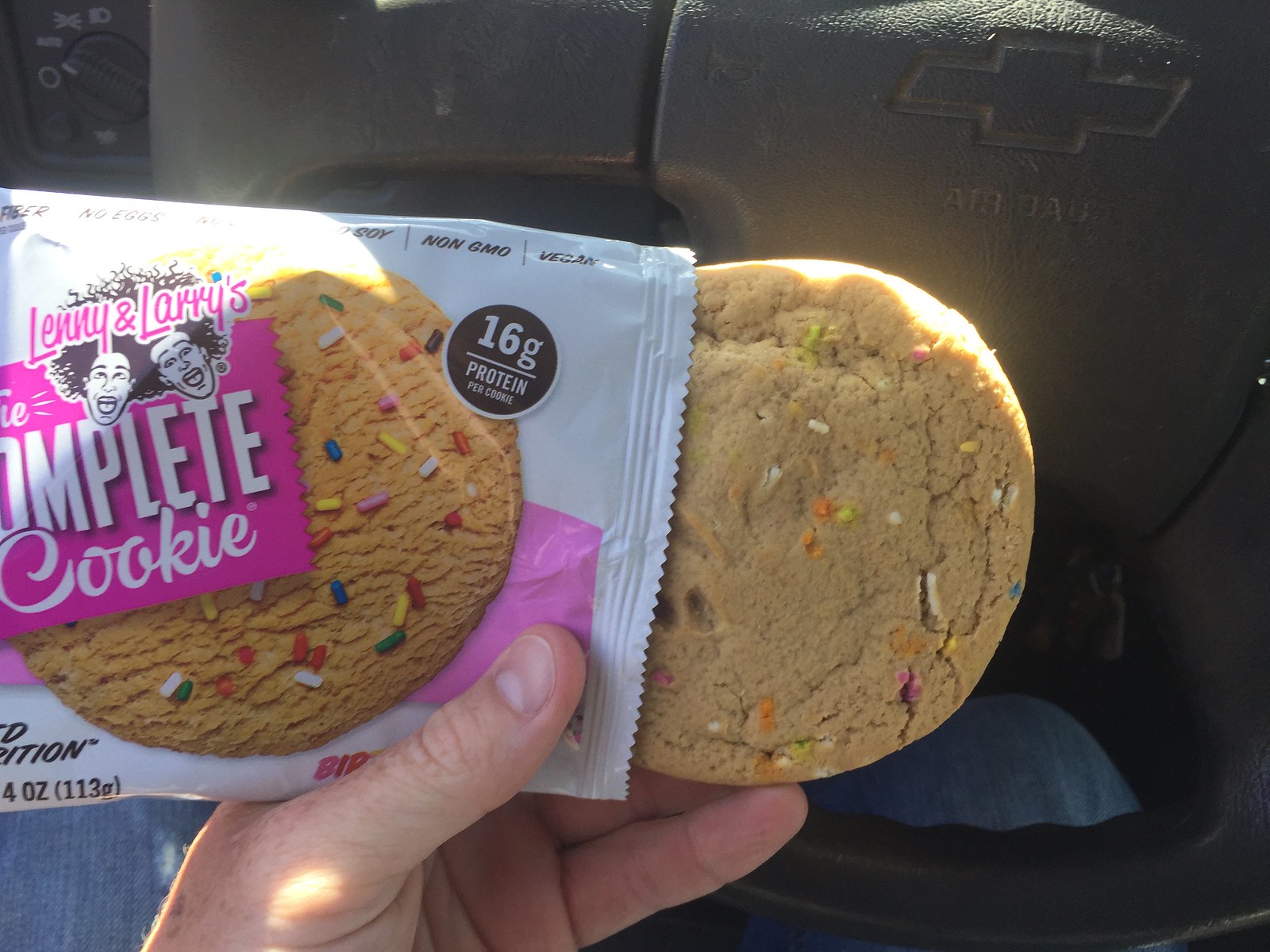A hand is prominently holding a mostly unwrapped cookie, revealing its tan surface adorned with colorful sprinkles. The wrapper, which remains on the left side of the cookie, features a white label against a purple background. The logo on the wrapper depicts two cartoon men with wild black hair and reads "Lenny & Larry's Complete Cookie," although the 'O' is missing in "Complete." Notably, it also mentions "16 grams of protein" in the upper right corner. Behind the hand, a car seat with the Chevy logo is visible in the background, along with a glimpse of the person's jeans in the lower left corner beneath their hand.